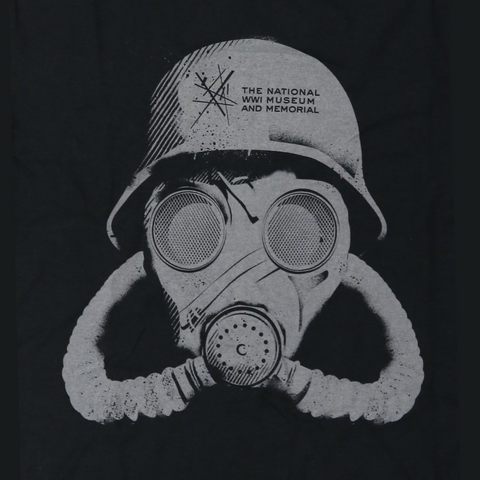This black and white illustration depicts a World War I-era gas mask adorned with a traditional metal soldier's helmet. The helmet prominently features the text "National WWI Museum and Memorial" on the front in black letters. To the left of this text, intersecting and diagonal lines create a shaded effect, adding depth and texture to the helmet. The gas mask below the helmet has two round eye lenses with crosshatching detail, adding a screened appearance. Horizontal lines accentuate the mask's mouthpiece, which is encircled by round holes. Two flexible, pipe-like tubes extend from the mouth area to the back of the mask, reminiscent of a double tank scuba regulator. The entire image is presented against a black background, highlighting the detailed illustration of the gas mask and helmet.